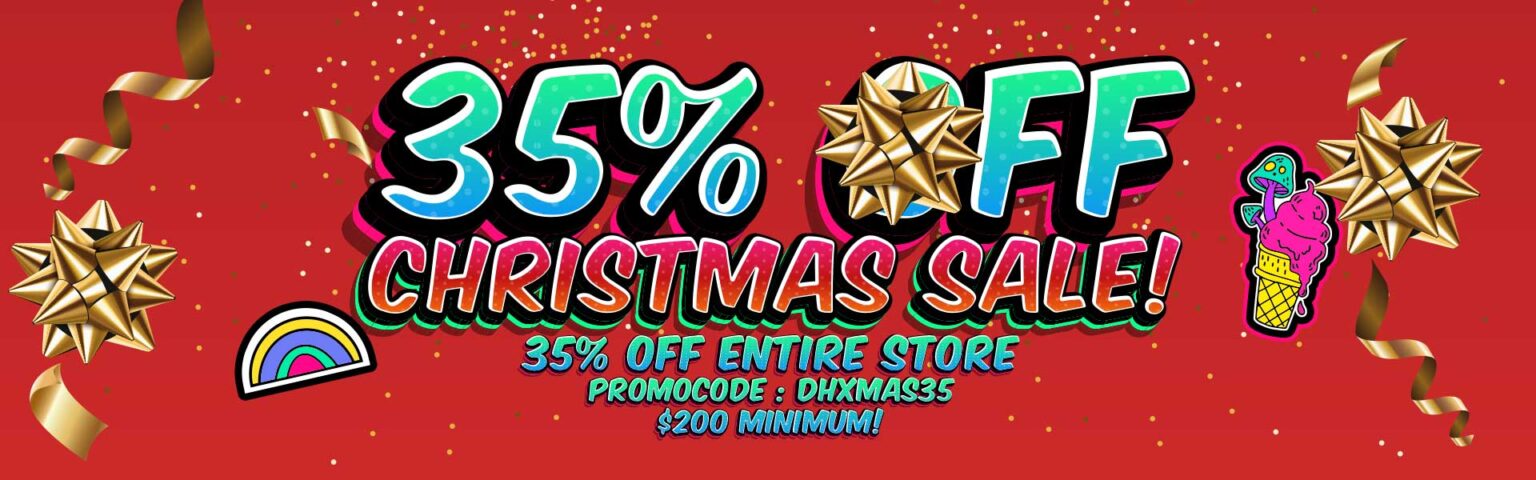This image depicts a vibrant advertisement characterized by its wide, horizontally rectangular format. The backdrop of the ad is a rich red color, adorned with gold confetti and streamers cascading from the top left corner and arching up towards the top right. Prominently displayed are large festive bows in a grey or gold hue, with one located at the bottom left, another centered over the "O" in the word "off," and another to the right.

Adding a whimsical touch, there are two clipart images: a rainbow positioned towards the bottom left and an ice cream cone placed near the center right. The ice cream cone features a yellow base with pink ice cream that gives the appearance of mushrooms growing from its sides.

The central text, placed prominently against this ornate background, reads "35% off" in an eye-catching and very large 3D font. Each numeral is shadowed by a substantial black outline with a white trim on top, filled with a gradient transitioning from green to blue at the bottom. Directly beneath, in equally large letters, the text "Christmas Sale" is displayed. This text uses a red-to-pink gradient and is highlighted with a black and then green outline.

Below the main promotional phrase, it states "35% off entire store" followed by a designated promo code, both centered for emphasis. At the very bottom of the ad, the terms "200 minimum" are clearly displayed, indicating the minimum purchase requirement for the discount.